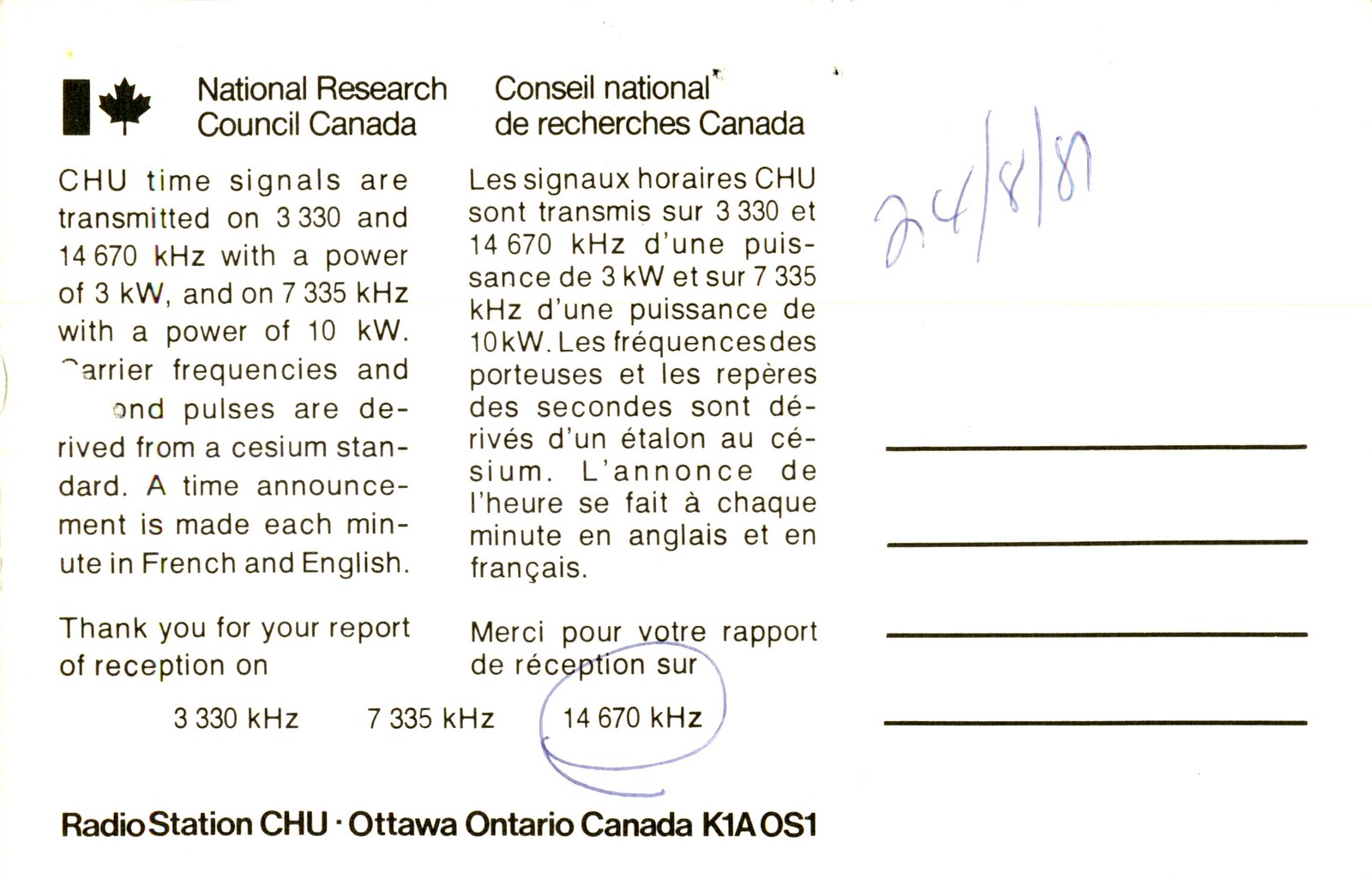The image displays a paper notice segmented into three columns. The left column features text in English, headed by the logo of the Canadian flag alongside the title "National Research Council of Canada." Beneath this, it states that CHU time signals are transmitted at 3,330 and 14,670 kHz with a power of 3 KW, and at 7,335 kHz with a power of 10 KW. It further details that the carrier frequencies and pulses are derived from a cesium standard, and time announcements are made in both French and English each minute. The text thanks the reader for their reception report on 3,330 kHz. In the right-side column, the identical information is provided in French. The bottom of the notice prominently features the black printed text: "Radio Station CHU, Ottawa, Ontario, Canada, K1AOS1." In the upper right-hand corner of the image, a date hand-written in ink reads "24-8-81." Adjacent to the French text are four horizontal black lines, but no further details are provided in this area.